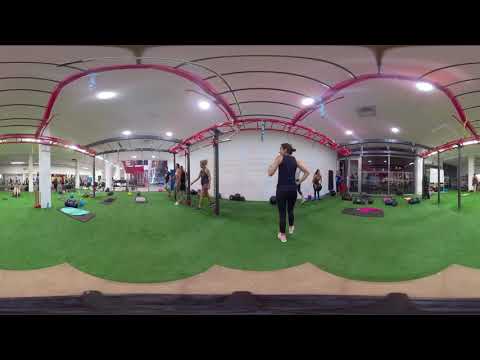The panoramic image captures an expansive indoor exercise studio with a green turf floor. The studio features an arched ceiling adorned with gray and red metallic elements, supported by white pillars and illuminated by fluorescent lights. At the center foreground stands a woman, seemingly the instructor, dressed in black tights and a purple tank top, jogging in place with pink sneakers. Surrounding her, against a white wall, are multiple participants in athletic wear, appearing to rest or await further instructions. Yoga mats of various colors, including blue and red, are scattered across the floor, though none are in use. To the right, a window and a doorway are visible, presumably leading to other areas of the gym. The image, bordered by black rectangles on the top and bottom, gives a wide, high-definition television-like perspective, emphasizing the vastness and energy of the bustling studio.